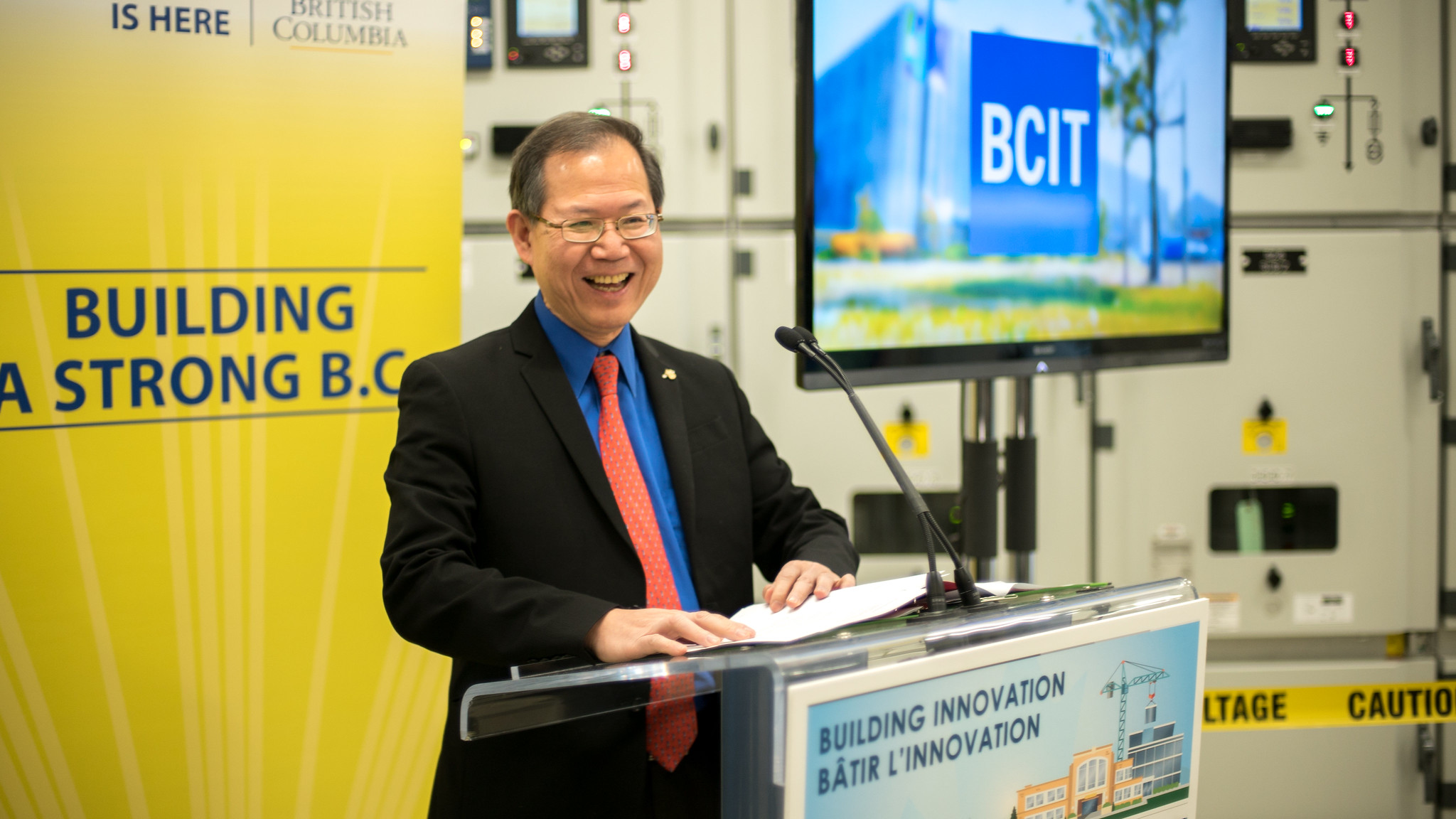This color photograph captures a close-up of an Asian man standing at a podium, giving a presentation at what appears to be a business conference in British Columbia. He is smiling and dressed in a black, unbuttoned blazer paired with a blue button-down shirt and an orange tie adorned with blue dots, tied in a Windsor knot. He wears glasses and has short, dark hair, slightly graying. A gold pin gleams on his blazer's lapel. The podium he stands behind is equipped with a microphone and features a prominent rectangular poster with an image of a building under construction, including a crane, and the text "Building Innovation" along with its French translation, "Bâtard l'Innovation."

Behind him, a monitor displays "BCIT" in large letters. To his right, a yellow backdrop reads "Building a Strong BCIT" in blue letters. The backdrop aligns with the overall theme of the event, emphasizing innovation in building. There are elements suggesting an industrial setting, including what appears to be caution tape with voltage warnings, indicating the presence of power equipment. The scene is likely part of an initiative or presentation related to advancements in construction or infrastructure in British Columbia.